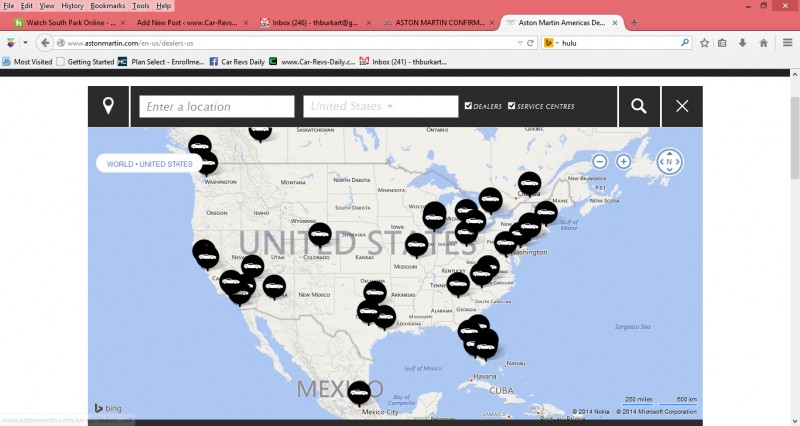This image displays the interface of a web browser. At the very top left, a menu bar with black text appears, featuring options such as File, Edit, View, History, Bookmarks, Tools, and Help. These words are set against a light pink background, which contrasts with the darker, hot pink background of the browser's title bar.

In the top right corner, typical browser control icons are visible: a white X for closing the window, a combined square and overlapped smaller square for resizing, and a dash symbol for minimizing.

Along the top tab bar, five tabs are open. The first tab, on the far left, is labeled "South Park Online." Next to it, the second tab reads "Cars Revs." The third tab appears to be for Gmail. The fourth tab is titled "Aston Martin," and the fifth tab reads "Aston Martin America's Deal."

Dominating the center of the image is a map displaying parts of the United States, Mexico, and Canada. Scattered across the map are various icons indicating the locations of Aston Martin cars.